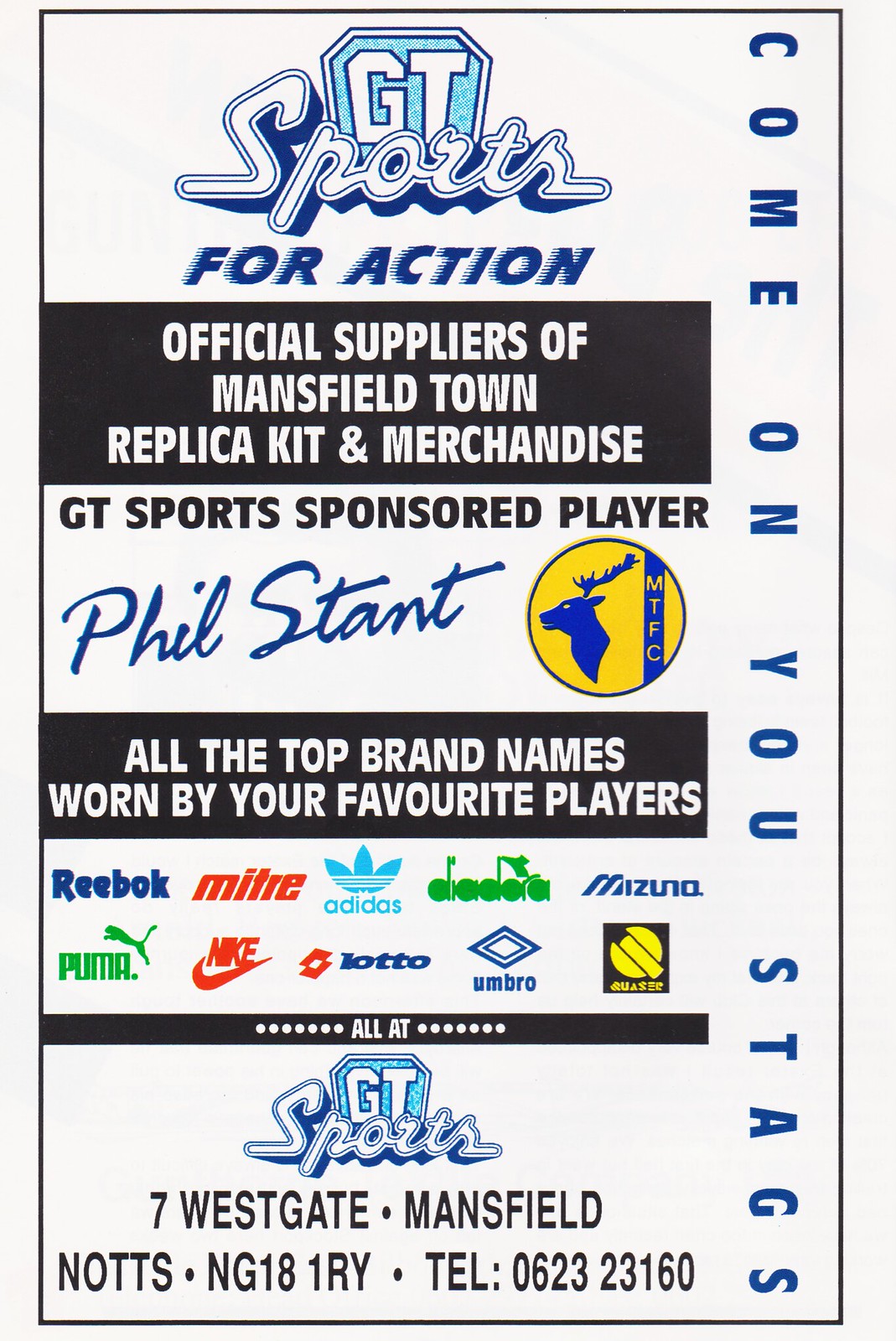This image depicts a promotional poster with a white background and a central black-bordered box. At the top, it prominently displays the title "GT Sports for Action" in a blue and white logo. Immediately below, with a black background and white text, it reads "Official Suppliers of Mansfield Town Replica Kit and Merchandise." Further down, it highlights "GT Sports Sponsored Player Phil Stant" in script. Adjacent to this, on the right, there is a yellow circle logo featuring an elk and "MTFC" inscribed, symbolizing Mansfield Town Football Club.

Underneath, another black rectangle contains the message "All the top brand names worn by your favorite players." Following this are logos of several prominent sports brands, including Reebok, Mitre, Adidas, Diadora, Mizuno, Puma, Nike, Lotto, and Umbro. The poster concludes with the contact details for GT Sports: "7 Westgate, Mansfield, Knotts, NG-18-1RY," along with a telephone number "0623-23160." On the right-hand side, vertically aligned in navy blue text, it encourages supporters with the phrase "Come On You Stags." The entire layout appears as if it might have come from a magazine, emphasizing its promotional and advertisement nature.